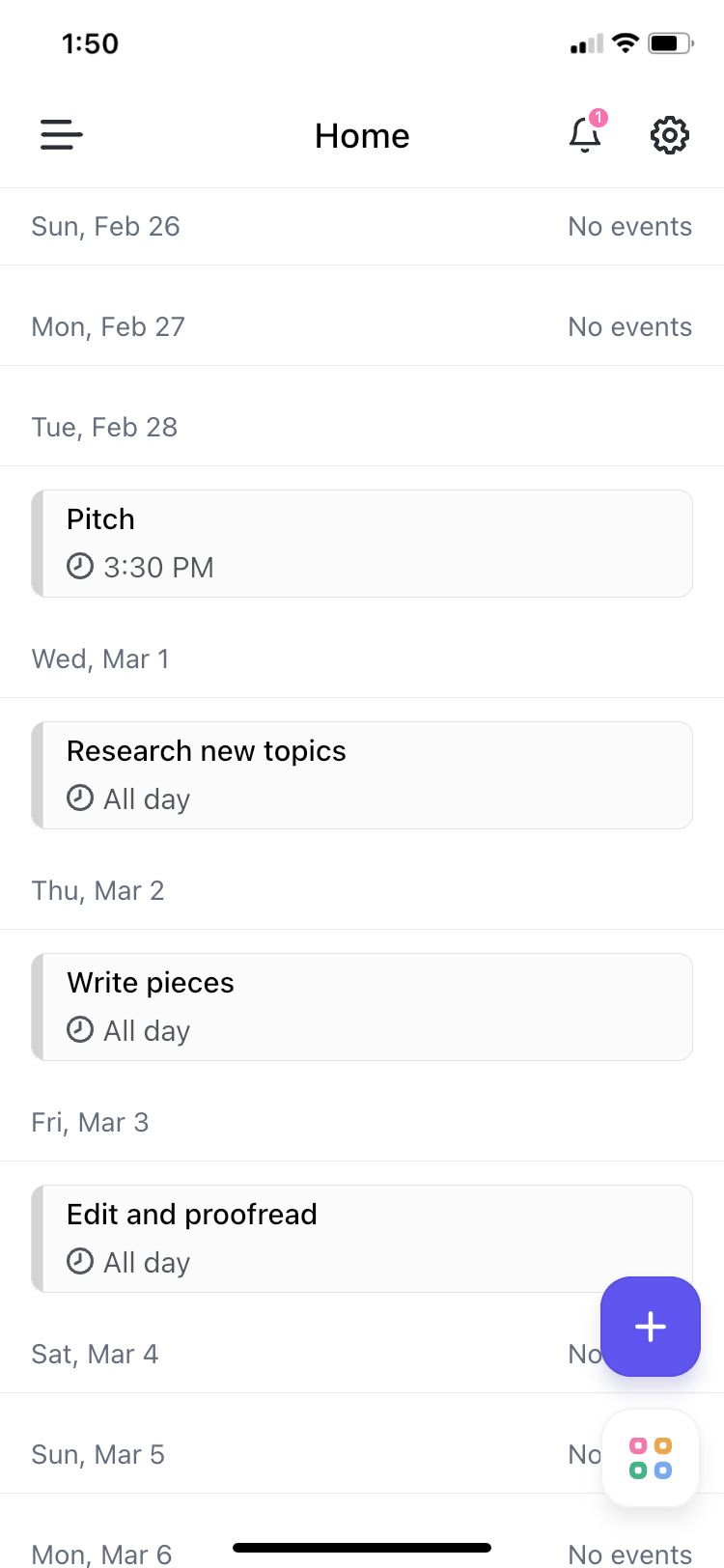Screenshot of a mobile day planner:

- **Top Navigation Bar:**
  - **Home Icon**
  - **Bell Symbol with Red Notification Badge**
  - **Cogwheel Icon**

- **Dates and Events:**
  - **Sunday, February 26:** No events
  - **Monday, February 27:** No events
  - **Tuesday, February 28:**
    - Event: "Pitch" at 3:30 PM
  - **Wednesday, March 1:**
    - Task: "Research New Topics All Day"
  - **Thursday, March 2:**
    - Task: "Write Pieces All Day"
  - **Friday, March 3:**
    - Task: "Edit and Proofread All Day"
  - **Saturday, March 4:** No events (noted with a blue box containing a plus symbol)
  - **Sunday, March 5:**
    - No events (with a white box featuring four different colored squares: red, yellow, green, and blue)
  - **Monday, March 6:** No events

- **Additional Details:**
  - **Time Displayed:** 1:50 PM (top left-hand corner)
  - **Platform:** Mobile device screenshot

The planner effectively lists scheduled tasks and events, highlighting certain dates with specific icons and color-coded boxes for quick reference.